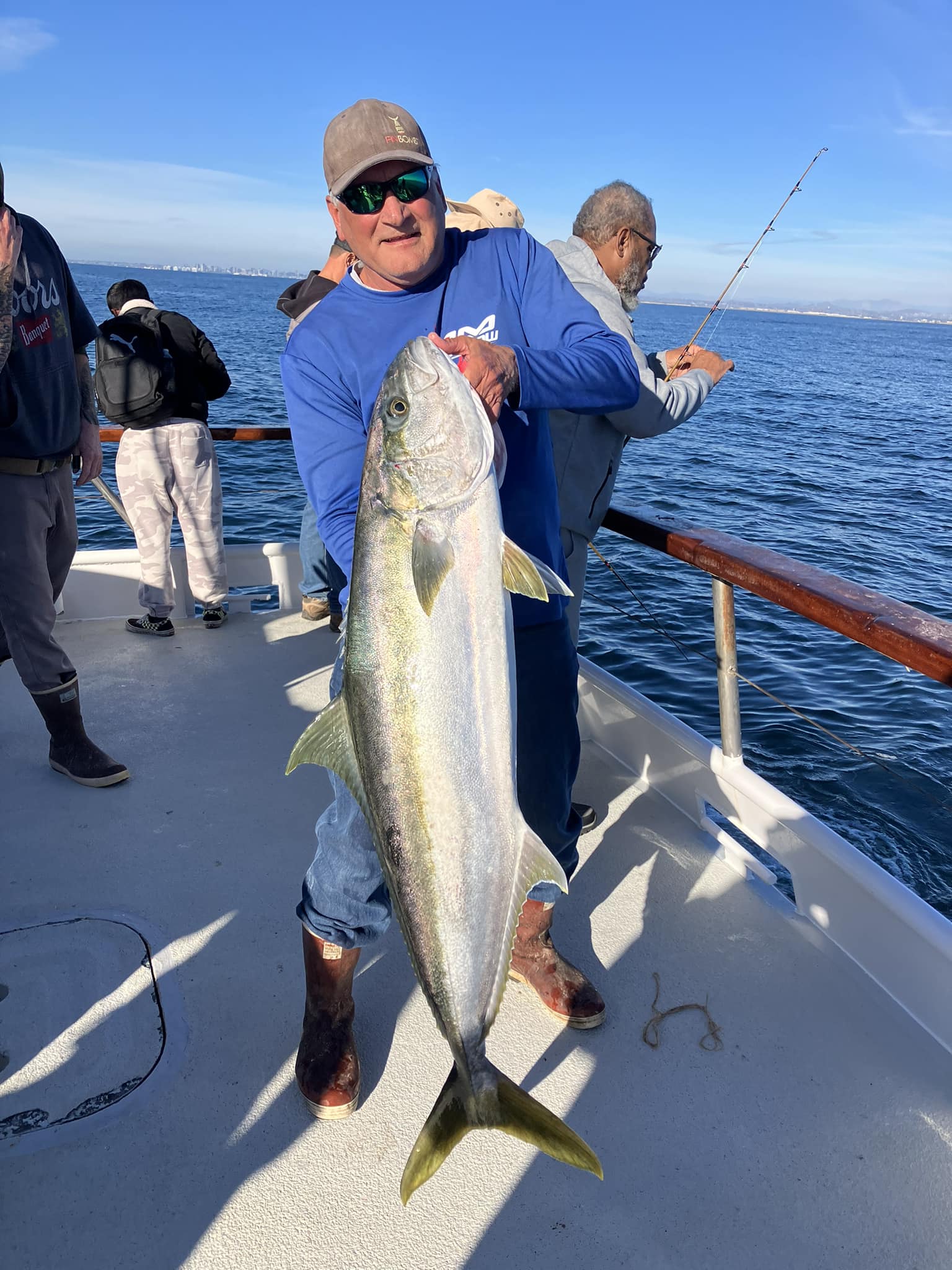In this vibrant photograph set against a clear blue sky and shimmering ocean, an older man, likely between 60 and 70 years old, stands proudly on the deck of a fishing boat. He is wearing a gray baseball cap and black sunglasses, along with a blue long-sleeve sweatshirt with indistinct white writing on the chest, blue jeans, and brown ankle-high boots. The centerpiece of the image is the massive fish he holds, measuring from the floor of the boat almost up to his neck, likely between four and five feet long. The fish has a striking appearance with a golden and black back, a white belly, and yellow fins. His left hand firmly grips the fish by its gills, prominently displaying its large black eye encircled by a lighter color.

To the right of the man is another older gentleman with short gray hair and glasses, holding a fishing pole and seemingly focused on the water. Behind them, partially visible, are the back of a man walking and another individual engaged in fishing. The boat's white structure with a brown banister wraps around the deck, framing the scene of an adventurous and fruitful fishing outing.